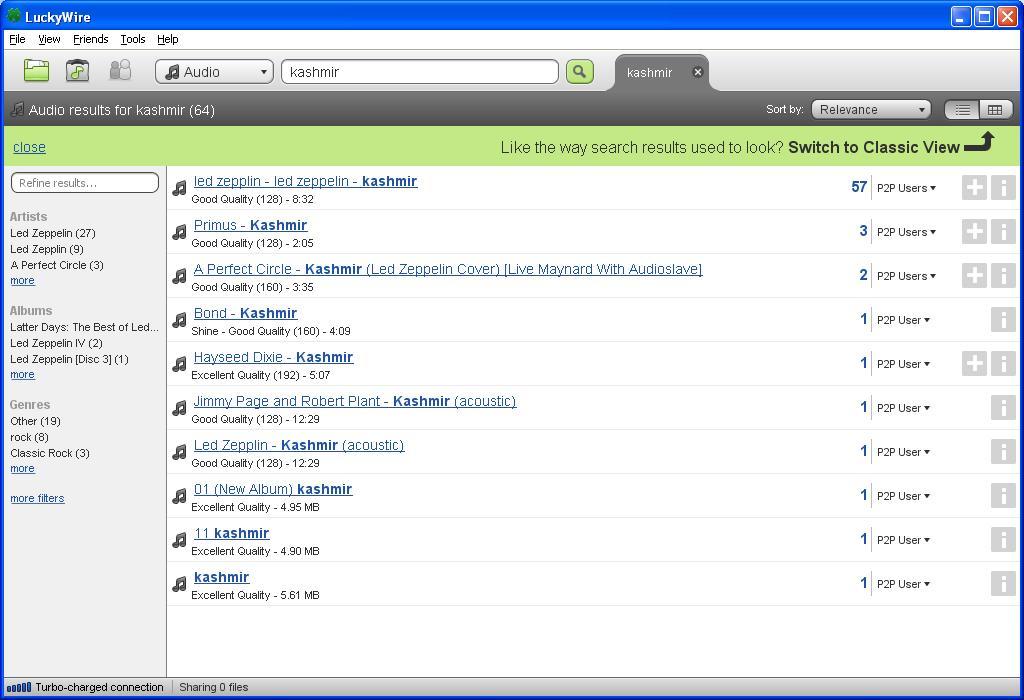This detailed image caption has been streamlined and formatted for clarity while maintaining all essential information:

---

Screenshot of the Luckywire application interface.

**Top Section:**
- A green four-leaf clover icon in the top left corner with the word "Luckywire" in white text on a blue background.
- Minimize, maximize, and close buttons in the top right corner.
- A white menu bar with black text featuring File, View, Friends, Tools, and Help.
- Below the menu bar, a gray toolbar with icons: a file folder, a music note inside a briefcase, and two user icons (one dark gray and larger, one white and smaller).

**Search Bar Section:**
- An options box with "Audio" selected, featuring dark gray musical notes and a drop-down arrow.
- A search bar with the word "Kashmir" inside.
- To the right, a green search button with a magnifying glass icon.
- Below the search bar, a dark gray tab labeled "Kashmir" in white text with a black circle and X icon.
- Main area beneath the tab states "Audio results for Kashmir (64)" in white text on light gray with gray musical notes.
- On the right, "Sort by" is followed by a selection box labeled "Relevance" and an oval with options for list or icon view.

**Left Sidebar (Light Gray):**
- A white selection oval labeled "Refine Results."
- Categories below:
  - **Artists:** 
    - "Led Zeppelin (27)", "Led Zepplin (27)", "Led Zeppin (9)", "A Perfect Circle (3)", "More" (blue, underlined).
  - **Albums:** 
    - "Latter Days: The Best of Led..." (black), "Led Zeppelin (4, 2)", "Led Zeppelin [Disc 3] (1)", "More" (blue, underlined).
  - **Genres:** 
    - "Other (19)", "Rock (8)", "Classic Rock (3)", "More" (blue, underlined), "More Filters" (blue, underlined).

**Main Content Section:**
- Large white background displaying search results.
- Each result line has dark gray music notes on the left with details in blue and black text:
  1. "Led Zeppelin - Led Zeppelin - Kashmir" (Kashmir in bold blue), "57" (bold on the right), "Good quality, 128 (8:32)".
  2. "Primus - Primus - Kashmir" (Kashmir in bold blue), "3" (bold on the right), "Good quality, 128 (2:05)".
  3. "A Perfect Circle - Kashmir" (Kashmir in bold blue), "Led Zeppelin cover [live Maynard with Audioslave]" (parentheses and brackets in regular blue), "2" (bold on the right), "Good quality, 160 (3:35)".
  4. "Bond - Kashmir" (bold on the right), "Shine - Good quality, 160 (4:09)".
  5. "Hayseed Dixie - Kashmir", "1" (bold on the right), "Excellent quality, 192 (5:07)".
  6. "Jimmy Page and Robert Plant - Kashmir" (Kashmir in bold blue), "Acoustic," "1" (bold on the right), "Good quality, 128 (12:29)".
  7. "Led Zeppelin - Kashmir" (Kashmir in bold blue), "Acoustic," "1" (bold on the right), "Good quality, 128 (12:29)".
  8. "Zero One - Kashmir" (bold blue), "New album," "1" (bold on the right), "Excellent quality, 4.95 MB".
  9. "11 - Kashmir" (bold blue), "1" (bold on the right), "Excellent quality, 4.90 MB".
  10. "Kashmir" (bold blue), "1" (bold on the right), "Excellent quality, 5.61 MB".
- Each result's right side features a drop-down for "P2P Users," some with icons for additional options (gray squares with white plus and "i" symbols).

**Bottom Section:**
- A gray bar with five blue lines (similar to signal strength indicators) labeled "Turbo Charge Connection," "Sharing 0 files."

---

This refined caption offers a clear and comprehensive understanding of the screenshot while maintaining essential details.